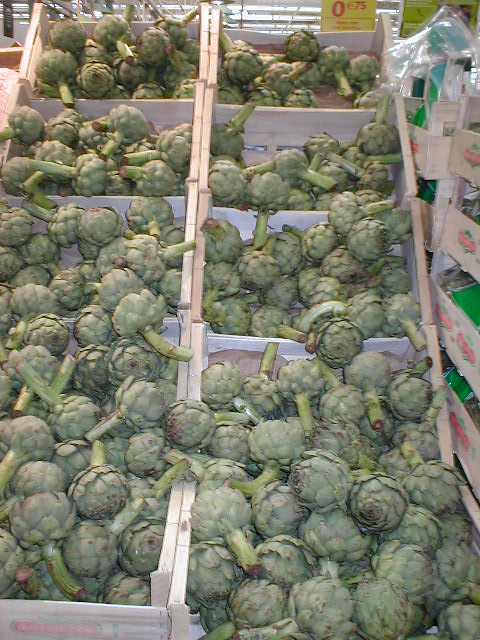The photograph captures an intricately arranged produce stand within a bustling supermarket or produce market. Eight wooden, basket-like boxes, stacked in a staircase formation, are filled to the brim with vibrant green Brussels sprouts. Each sprout is rounded, similar in shape to small heads of cabbage, and has a short stem, about four or five inches in length. These sprouts, with their tightly layered leaves, resemble miniature armadillos. Above the neatly organized stacks, a yellow sign prominently displays the price, indicating 0.75 euros per unit. Adjacent to the Brussels sprouts are additional boxes containing a variety of other vegetables, adding to the rich tapestry of fresh produce on display.